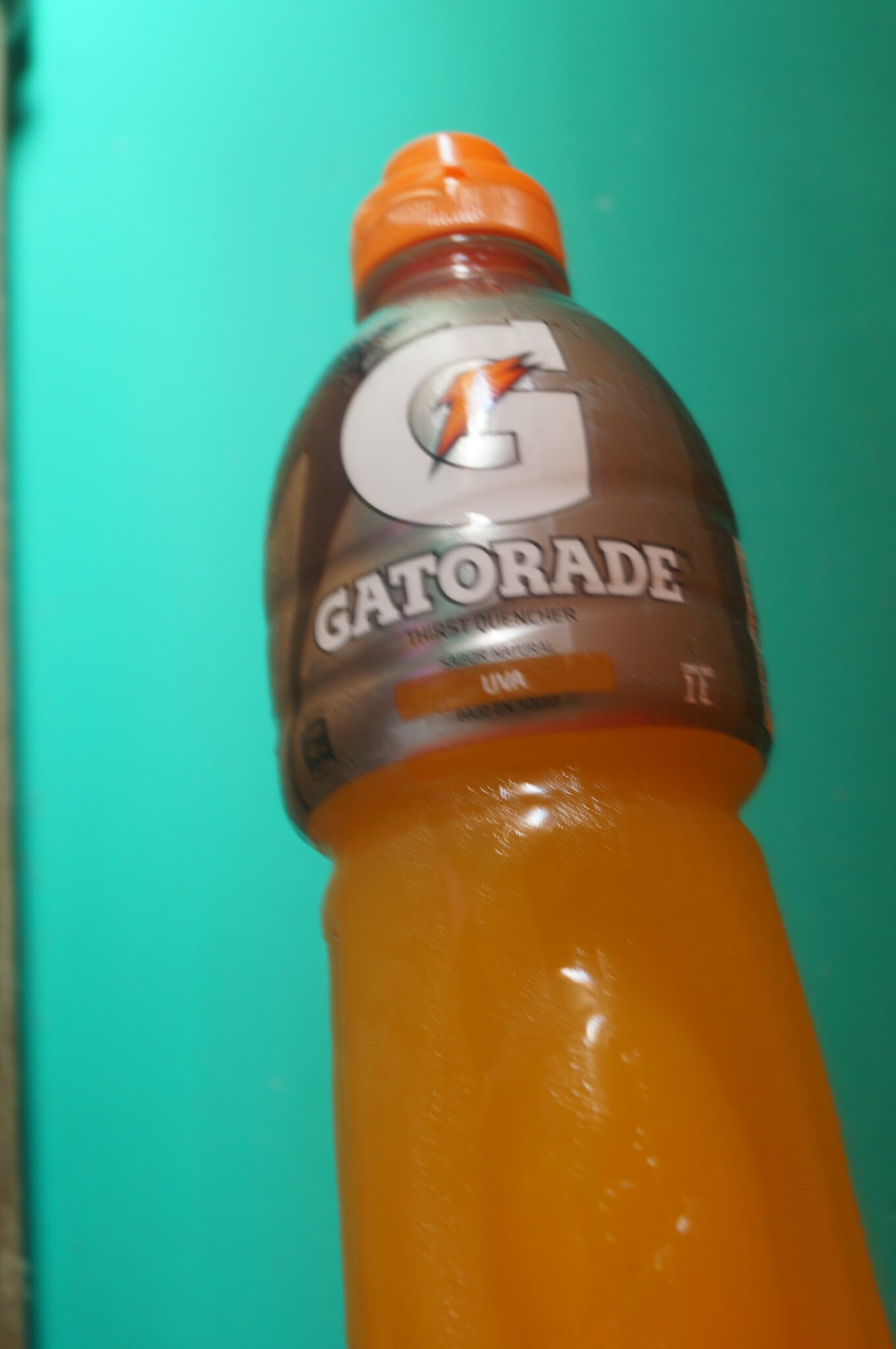This image is a detailed color photograph of a plastic sports bottle of orange Gatorade, set against a bright teal backdrop. The clear bottom half of the bottle reveals the vibrant orange liquid inside, resembling the hue of orange juice. The label, primarily gray, prominently features the classic Gatorade branding. At the top, beneath a large white "G" with an orange lightning bolt, "Gatorade" is spelled out in bold white bubble letters. Below that, thinner black text reads "Thirstquencher." Additionally, an orange and gray section of the label contains the abbreviation "UVA" in white letters. The bottle is topped with an orange squeeze cap, completing the sports bottle appearance. On the left edge of the image, there is a sliver of gray, possibly part of another object or the photograph's border.